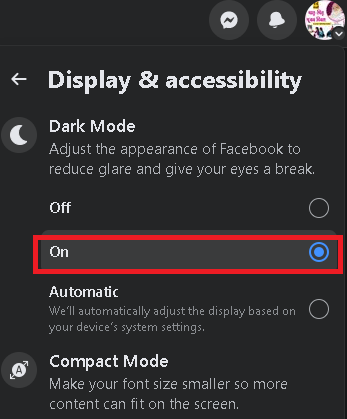In this image, we can see a settings menu, specifically under the "Display and Accessibility" section. The background is predominantly black with white text, indicating that dark mode is active. 

At the upper right corner of the screen, there are three icons: one resembling the Facebook Messenger icon, another resembling a notifications bell, and the last one depicting the user’s profile picture. 

Just below these icons, the section header "Display and Accessibility" is visible, accompanied by a back button for navigation.

The first option under this section is "Dark Mode," which includes a description reading, "Adjust the appearance of Facebook to reduce glare and give your eyes a break." There are toggle options labeled "Off" and "On," with the "On" option currently selected, explaining why the background is black.

Beneath the dark mode settings, there is an "Automatic" option, which states, "Will automatically adjust the display based on your device's system settings."

Further down, we see "Compact Mode," which offers the option to make font sizes smaller so more content can fit on the screen.

In the image, a rectangular highlight around the "On" setting for dark mode emphasizes its selection, indicating it has probably just been toggled on by the user.

Overall, this image shows a straightforward settings menu focusing on display and accessibility options on Facebook, with the main feature being the dark mode setting.